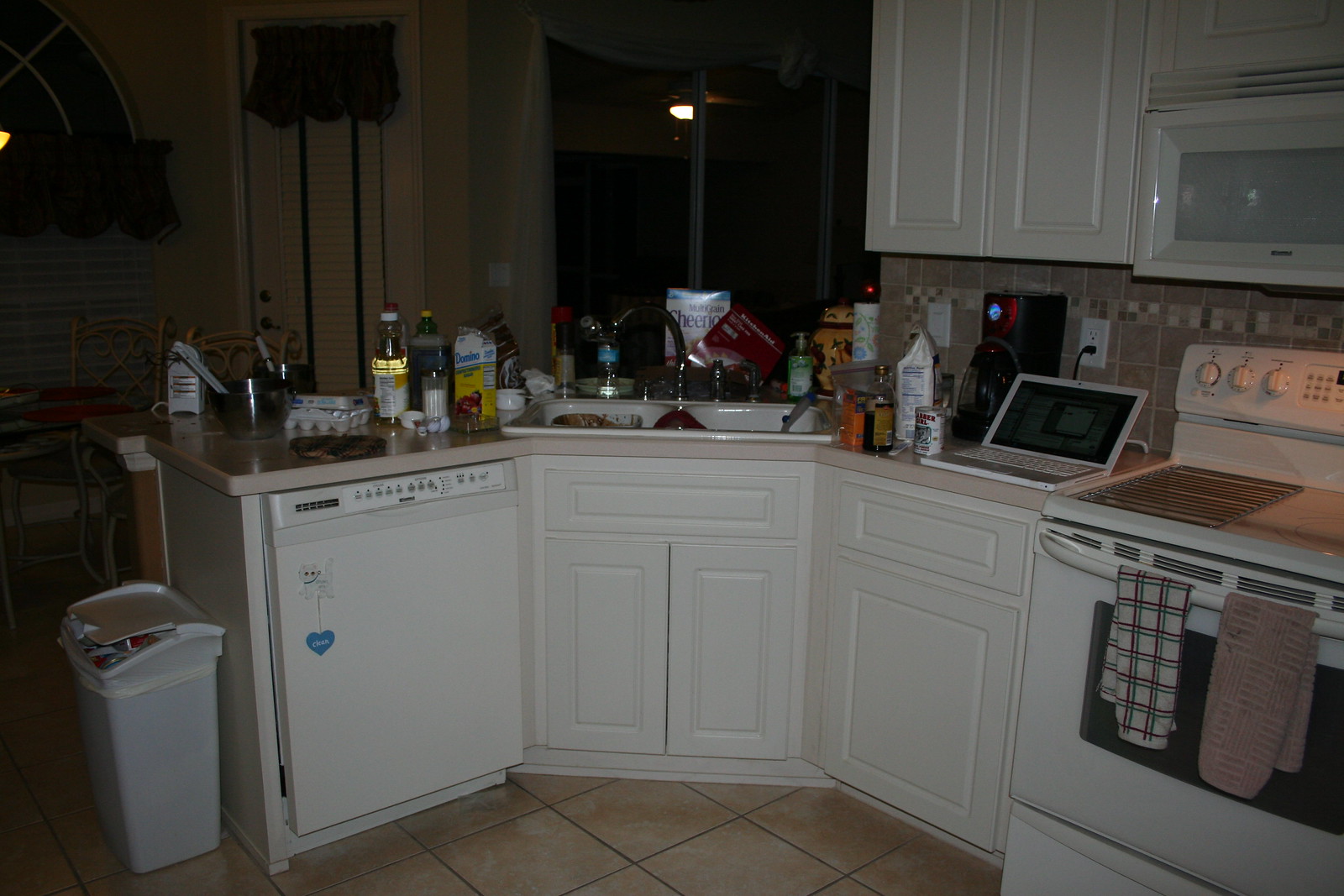The photograph, captured in color and in landscape mode, depicts a kitchen interior at home with dim lighting. On the right-hand side, a white stove is visible, adorned with two towels hanging from the oven door rail; the towel on the right features a light pink pattern, while the towel on the left displays a flag-like design with green and red stripes on a white background. Above the stove, a white microwave oven is situated.

To the left of the stove, a countertop holds a white laptop plugged into an outlet, accompanied by a can of baking powder, a chrome coffee maker, a bag of unidentified ingredients, and a half-full bottle containing a dark liquid. Above this counter space, a white double cabinet is mounted.

Further left, a white kitchen sink with a chrome faucet is observed, cluttered with dirty dishes. Positioned behind the sink is a box of Multigrain Cheerios. Adjacent to the sink on the left side is a white dishwasher. Beneath the sink are two white cabinets, while the countertop above the dishwasher holds various items, including a carton of eggs, a bottle of cooking oil, a box of Domino's sugar, and other indistinguishable objects due to the low light.

On the far left, a white plastic trash can with a lid, filled with trash, completes the scene. The clutter and everyday kitchen items lend an authentic lived-in feel to the space.